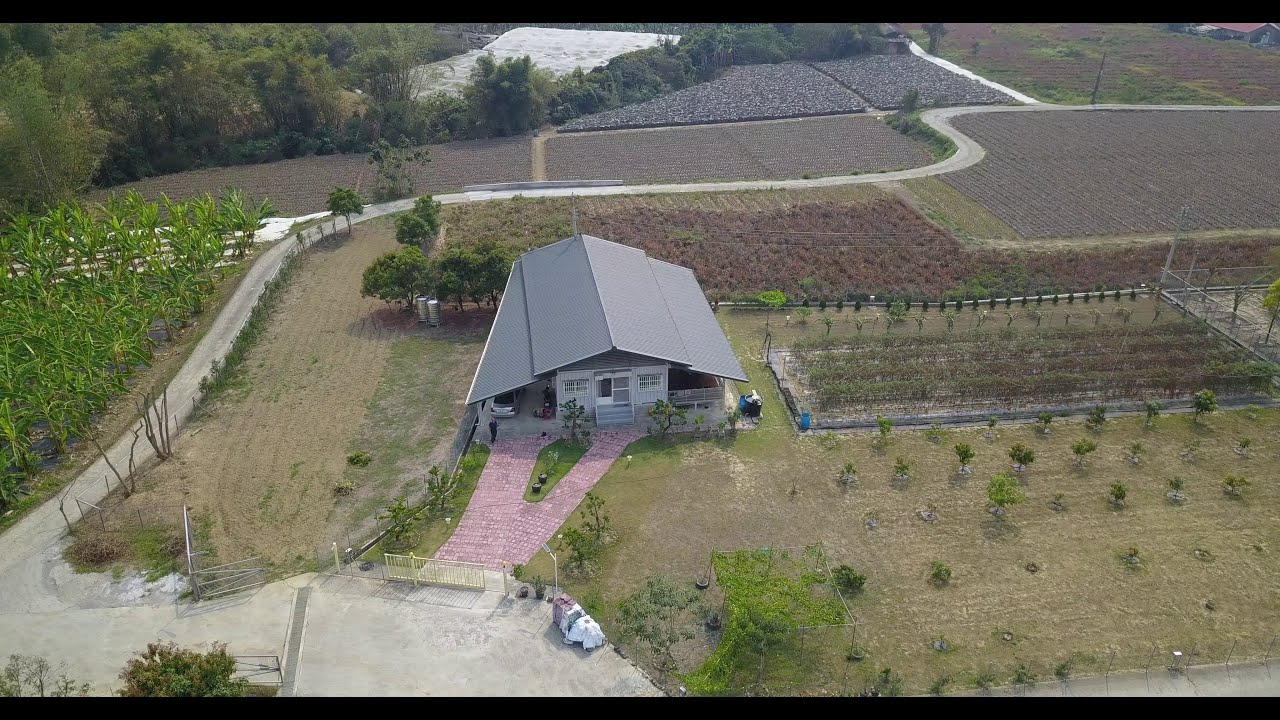This aerial view features a farmhouse with a prominent gray triangular roof at the center, surrounded by well-organized garden areas. A pathway curves around the front of the building, connecting to a smaller road in the lower left. To the left of the image, lush green vegetation occupies a neatly sectioned field, while behind the house, there are fields with red-colored plants and others where crops are either still growing or yet to sprout. Additionally, a silver sedan is parked next to the building, with a person standing nearby. The garden areas are divided into various shapes and sections, planting different types of vegetation, creating a vibrant mosaic of colors and textures. Towards the back of the property, several trees provide a natural border to the landscape. Overall, the scene showcases a meticulous and well-maintained agricultural setting.